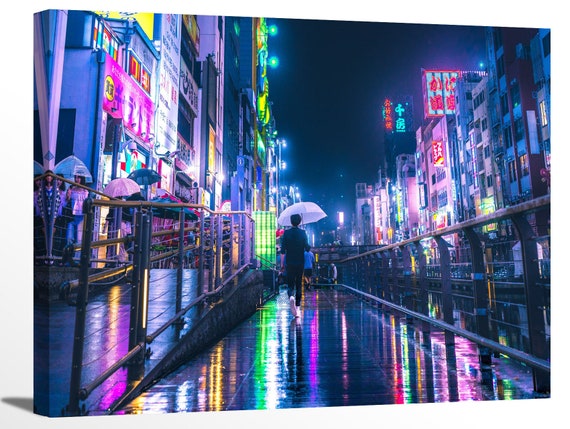In this vivid, full-color nighttime photograph, we see a bustling city street illuminated by an array of neon signs in colors ranging from pink, purple, and blue to neon green, yellow, and gold. The setting is a rainy night, with wet pavement reflecting the vibrant lights of tall buildings on either side. At the center of the scene, a person dressed in jeans, a dark shirt, white shoes, and holding a white umbrella walks away from the viewer. To the left of this figure, several other pedestrians with umbrellas approach, navigating a sidewalk or a ramp flanked by railings that suggest a descent to an underground area. The image appears on a boxy canvas, with a small light border and a shadow visible in the lower-left corner. The signs on the buildings, displaying text in an unreadable language, add to the urban mystique. Despite the downpour, the atmosphere is lively and colorful, capturing the essence of city life after dark.